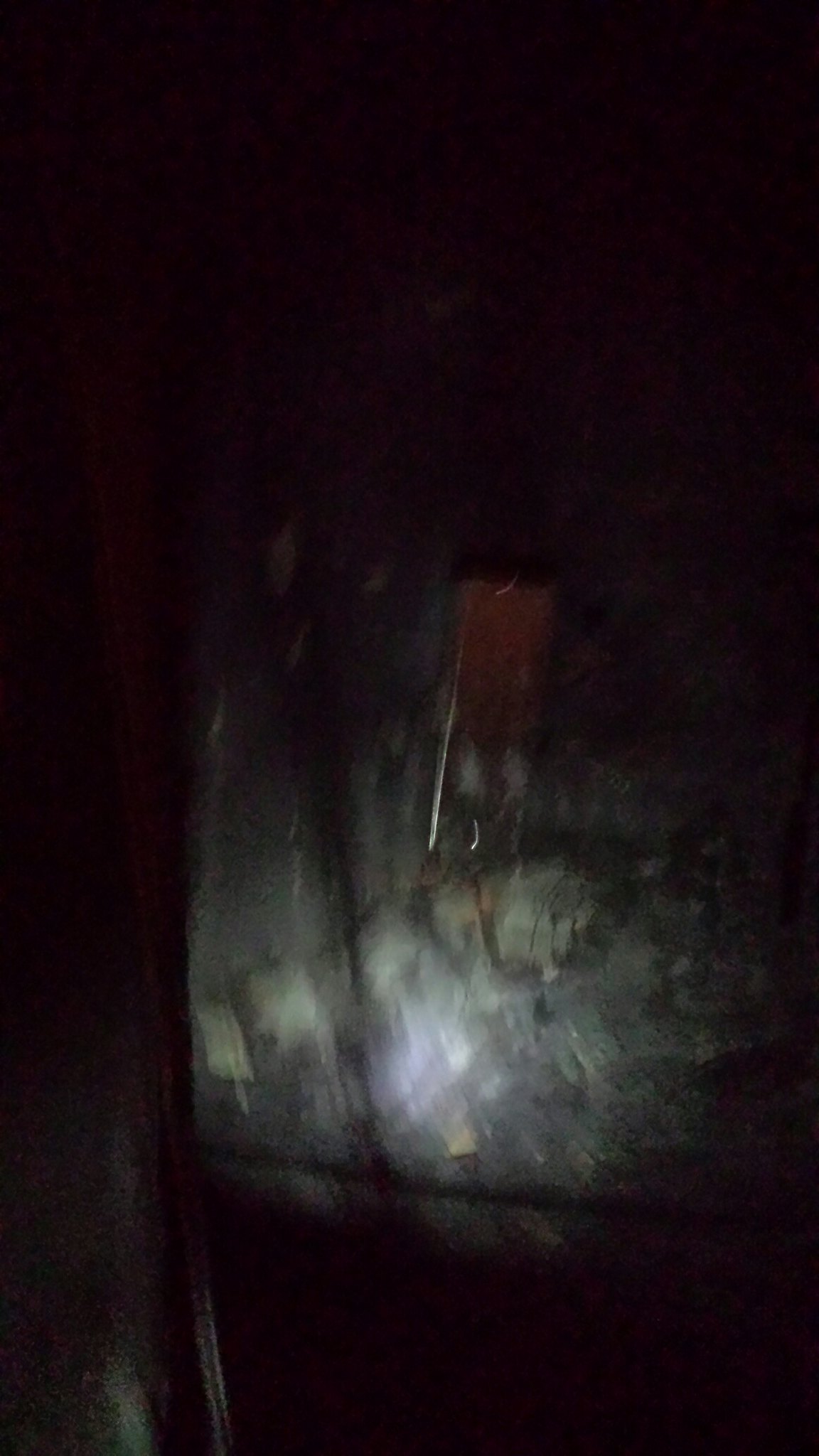In the image, there is a predominantly dark area with patches of reflected light, showcasing hues of gray and black. The surface appears to be slick and oily, and a silver line is noticeably dripping from the top toward the bottom. Additionally, there are visible streaks of gray that underscore the reflective quality of the material, which resembles an unspecified type of metal. The overall image is somewhat blurry, suggesting that the object might be in motion.